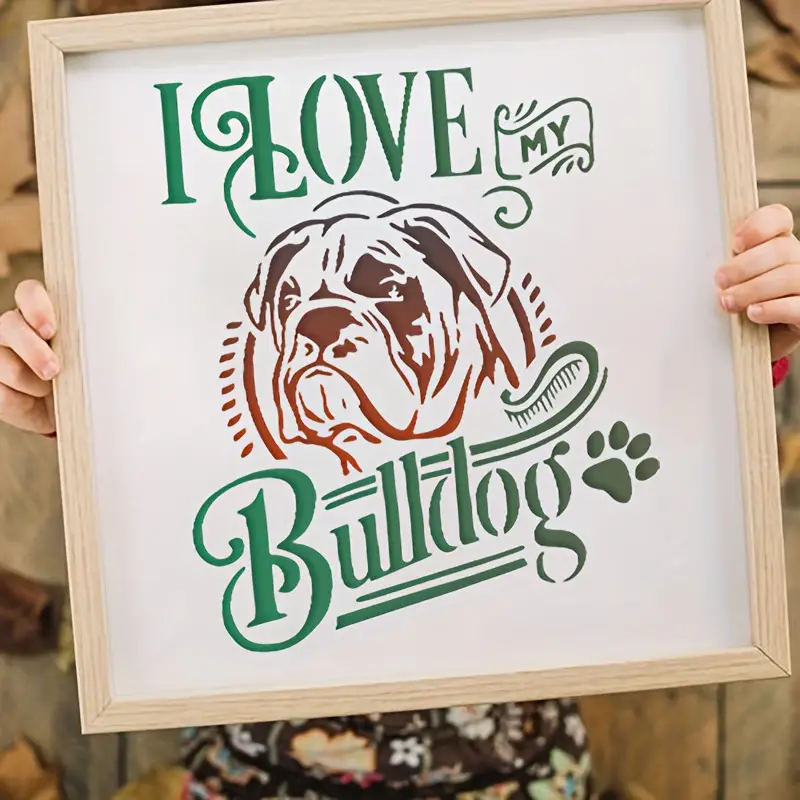The image captures a light-colored tan wooden frame being held up by a person, revealing just their fingers gripping the sides and a glimpse of their lower body dressed in black attire with floral patterns. The frame's inscription, crafted in a cursive green font, reads "I love" at the top, with "my" written in a cute banner style in the middle, and "bulldog" at the bottom, accentuated by a green paw print to the right. Inside the frame, a depiction of a bulldog's face is rendered as an outline in a brownish-red gradient. The background within the frame is white, and the overall setting, slightly blurred, shows an indoor scene with a wall behind the person.